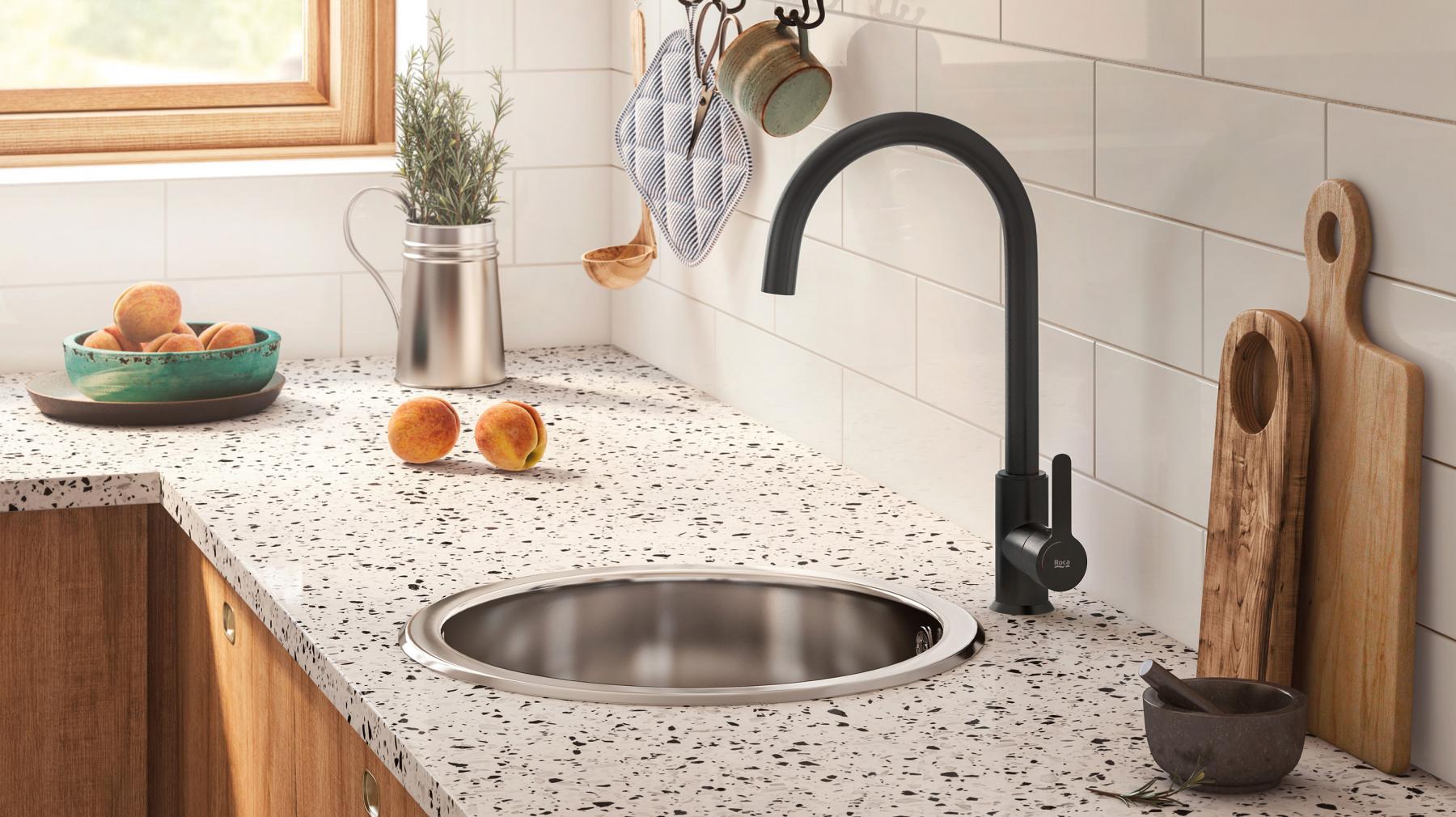The image showcases a cozy corner of a rustic kitchen counter with detailed elements. Centered in the scene is a plain silver sink with a distinct, modern black faucet shaped like a swan's neck. The countertop, speckled in white and black, spans the lower half of the image, contrasting with the warm, wooden cabinets beneath that have stainless steel recessed handles. The backsplash is a clean white tile that climbs halfway up the walls. 

To the left of the sink near the window, a green jade-colored bowl perched atop a smaller one cradles a bounty of peaches, with two more peaches casually placed on the granite counter. The window, trimmed in wood, allows bright sunlight to filter in, hinting at a lush, green outdoor scene. A silver canister, brimming with rosemary, adds a touch of greenery and aroma to the setting.

The scene is complemented by a variety of kitchen utensils and decor: a bamboo spoon, a soup ladle, an oven mitt, a pair of scissors, and a measuring cup hanging on the wall. By the window, there's also a mug with more rosemary. On the right, a wooden charcuterie board and a gray mortar with a pestle rest near a black bowl. This kitchen corner, bathed in natural light, melds both modern and traditional elements, creating a warm and functional space.